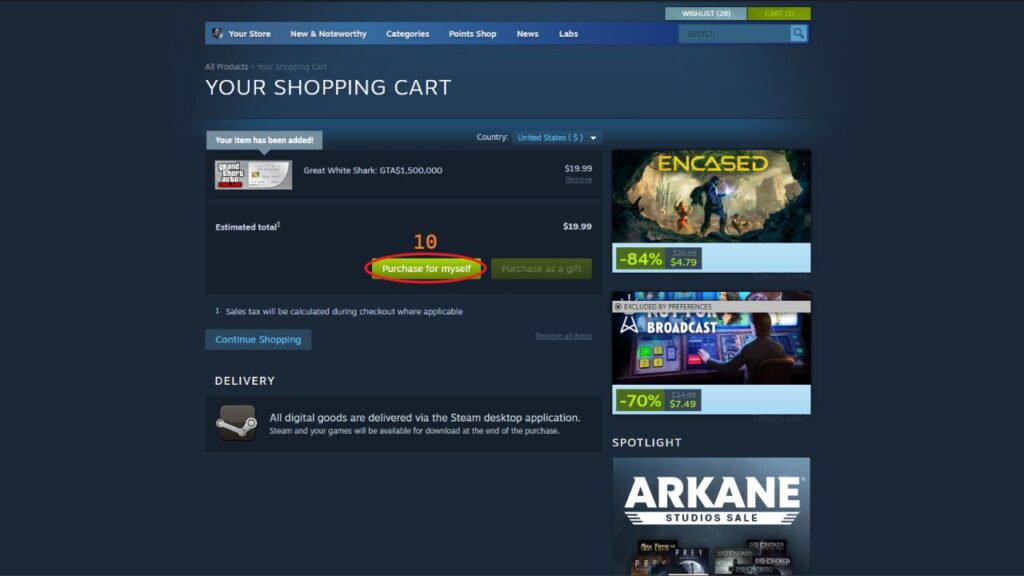The image depicts a web page interface predominantly colored in dark navy blue. At the top of the page, there is a navigation bar featuring several options written in white font, including "Your Store," "New and Noteworthy," "Categories," "Points Shop," "News," and "Labs." Additionally, "Watch List" is shown in gray, while the "Cart" button is highlighted in green. Adjacent to these options is a search bar accompanied by a magnifying glass icon, colored in a darker shade of blue.

A pop-up notification indicates that an item has been added to the cart, specifically the "Great White Shark" in the game "Grand Theft Auto," offering 1.5 million in-game currency for $19.99. The estimated total is displayed, and purchasing options are provided: "Purchase for Myself" is circled in a prominent red bar, while "Purchase as Gift" is grayed out. Additionally, there is a "Continue Shopping" option available for further browsing.